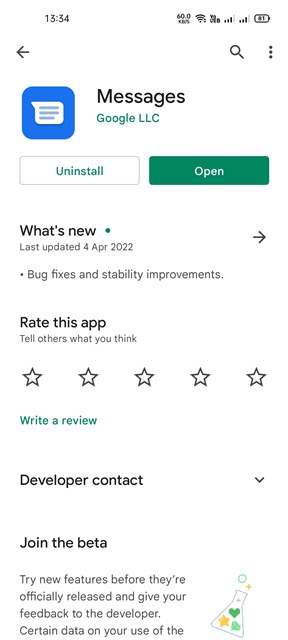A detailed view of an iPhone screen displays an app information page in the Google Play Store interface. The status bar at the top shows the phone time as 1:34 PM, with the date in a 24-hour format (13:34). It also indicates a Wi-Fi connection with full bars, a cellular connection with moderate strength (around three bars), and a battery level at 81%.

Below the status bar, the interface starts with three dots and a search magnifying glass on the left. The main content area features a prominent blue box displaying the app icon resembling a folded paper, alongside app details such as "Messages by Google LLC." The interface presents options in green and white boxes, offering to "Uninstall" the app or "Open" it, suggesting the app is newly installed.

Further down, under a "What's new" section highlighted, the text notes the latest updates dating from April 2022, including 'bug fixes and stability improvements' in black font. An arrow directs users to additional details.

Next, a "Rate this app" section appears, encouraging users to leave feedback via a 5-star rating scale, which currently shows no selected stars. Below that, a "Write a review" option is highlighted in green.

The screen also includes a "Developer contact" section that can be expanded for more information, indicated by a downward arrow. At the bottom, a 'Join the beta' section invites users to test new features before their official release. This area is marked by an icon resembling a flask with a yellow star, green heart, blue bubble, and a plus sign emerging from it, indicating experimentation and feedback opportunities.